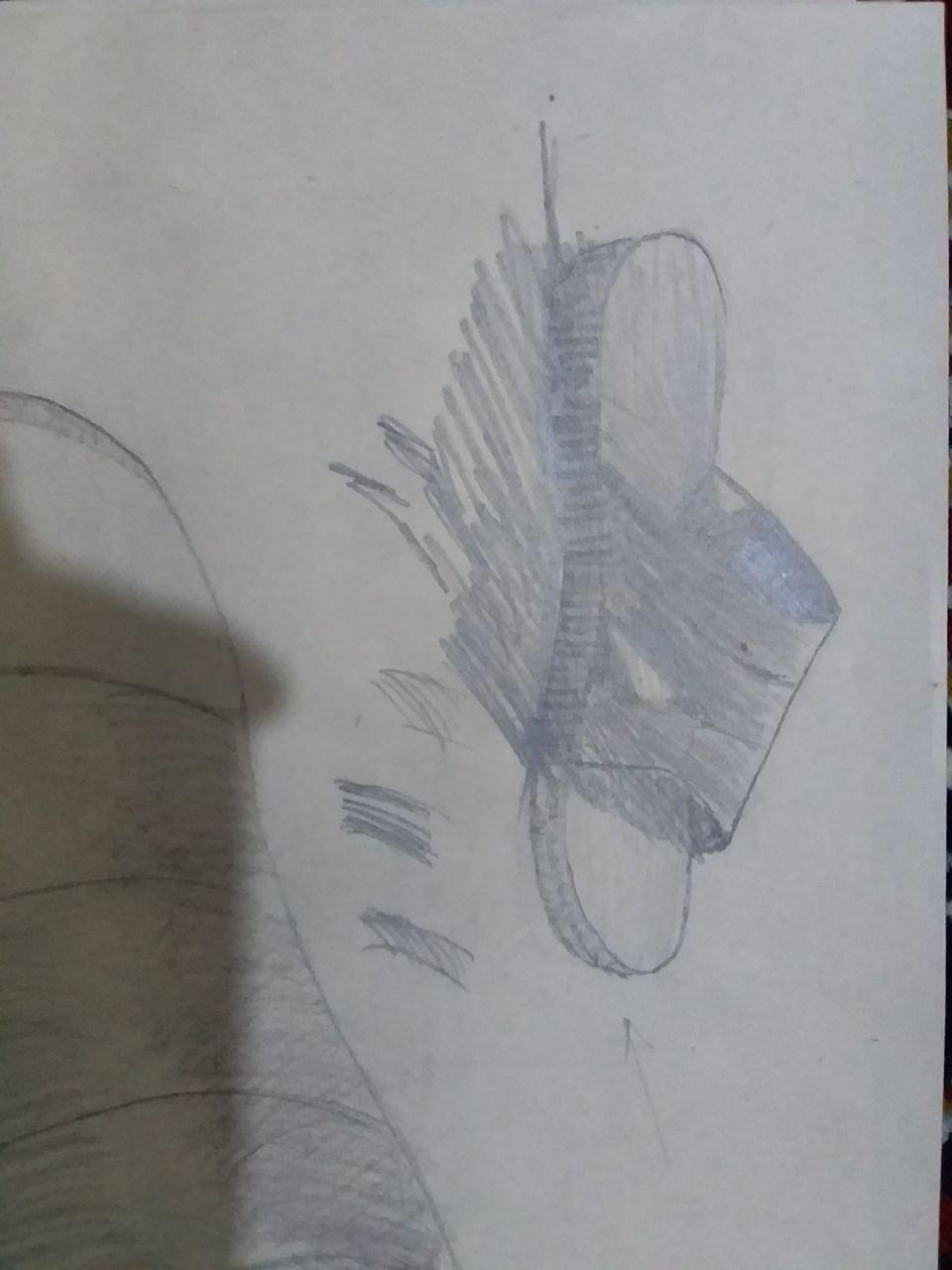A vertical pencil drawing of a Nike sandal occupies the majority of an off-white sheet of paper, which is about 50% taller than it is wide. The sandal, identifiable by the Nike swoosh, is positioned facing downwards, resembling 6 o'clock on a clock face. It features an open toe and a thick sole, with the strap displaying a small gap for ventilation. Shadowing from the sandal is evident to its right side, our left. In the lower left corner of the image, there's a detailed drawing of a thumb, depicted around two-thirds up the image and covering approximately two-thirds of the thumb. This thumb appears to be holding the page down. Additionally, another shadow extends diagonally from the center left to the bottom left of the image. Overall, the detailed shading particularly emphasizes the sole and the contours of both the sandal and the thumb.